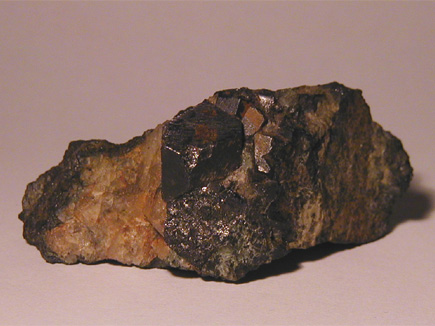This is a detailed color photograph focused on a uniquely textured rock mineral. The rock features a complex combination of colors including black, gold, beige, and clear white, with some parts appearing opaque. Central to the rock is a shiny portion that exhibits variations in color and texture. To the right of the center, there are small, irregularly shaped, light beige elements arranged vertically. Adjacent to this section is a large, dark brown or blackish oval shape. The left edge of the rock displays a beige-gold tone with a darker edge, while the right side transitions into dark gray tones. The overall structure of the rock is shallow in height and wider at the base, showcasing different shapes and specks throughout. The background is a faded reddish beige, and the image is small, approximately three and a half by three and a half inches, with no visible identifying information such as a date, name, or presence of people. The style of the photograph is highly detailed and realistic, capturing the intricate natural beauty of the mineral.